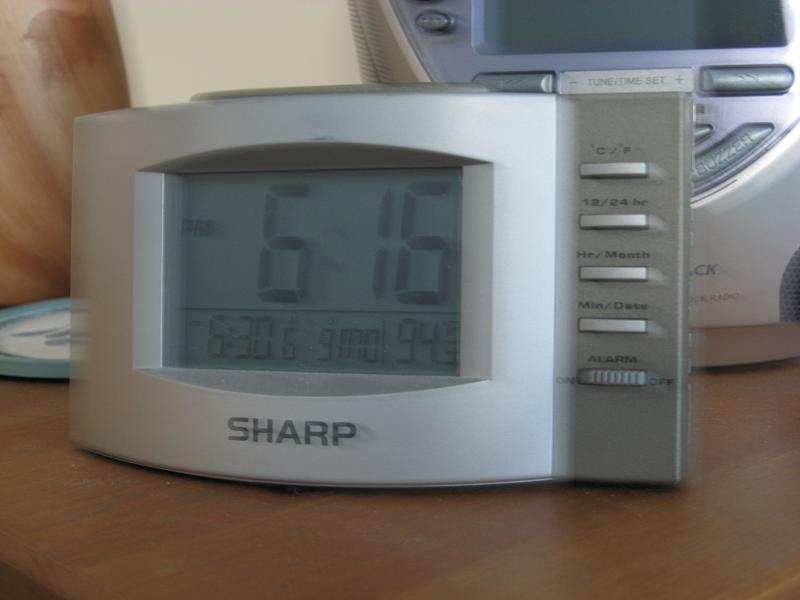This image features a Sharp brand rectangular desktop alarm clock with a rounded face. The digital LCD display shows the time as 6:16, and at the bottom, it indicates an alarm set for 6:30, the temperature at 94.3 Fahrenheit, and a date that reads "9 months." The right side of the clock houses a darker gray control panel equipped with buttons and a toggle switch for turning the alarm on and off. The clock is placed on a wooden table. Directly behind it sits a larger gray boom box with a blue face and a digital screen that is currently off, partially obscured by the smaller alarm clock in front.